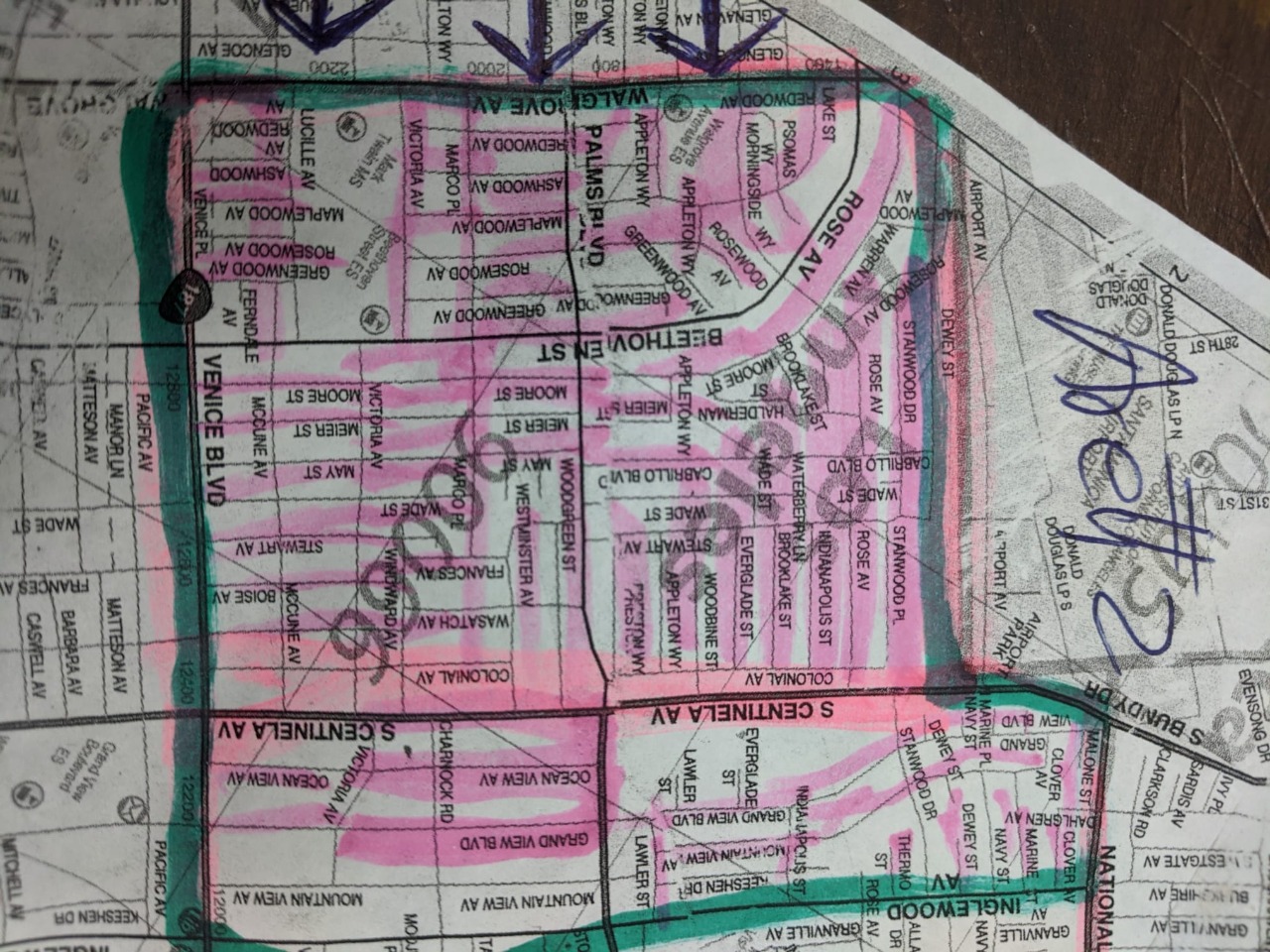This rectangular, horizontally longer photo prominently features an old, aged street map that occupies approximately 90% of the image. The map, characterized by a worn whitish-gray color, displays numerous outlines and handwritten annotations across its surface. In the upper right corner, a small triangular section of a dark brown wooden tabletop or countertop is visible.

The street map includes several distinct sections and markings. In one squared-off area, outlined in green marker, three black arrows point towards the top of the section, denoting specific areas of interest. Within this section, various streets are identified, including Venice Boulevard running north to south, and Rose Avenue and Beethoven Street running east to west. Below these, South Centinella Avenue also runs east to west. The bottom of this marked section features the word "Englewood."

The upper left corner of the map is notably worn, with the black print faded and barely legible, though the upside-down word "Grove" can be discerned. In the lower right corner, "South Bundy Drive" is clearly printed in black, running horizontally across the map.